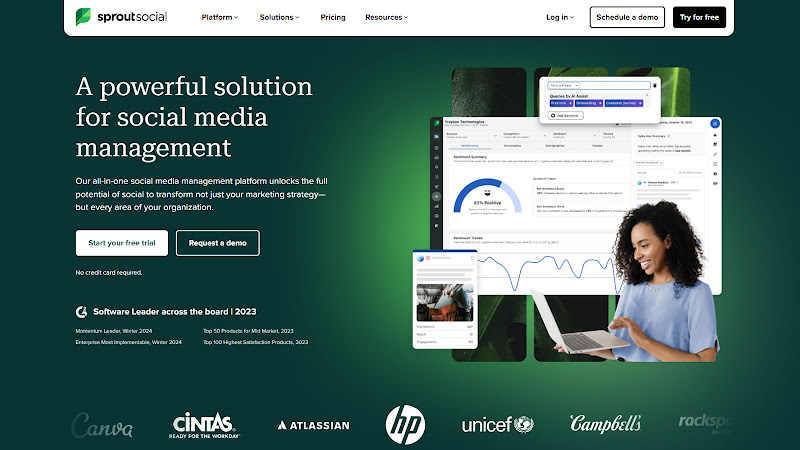The image showcases the homepage of the Sprout Social website. The screen primarily features a dark green background with a lighter green accent in the middle, complemented by white text. At the top of the screen, a white header bar displays "Sprout Social" in bold black text. To the right of the logo, the menu options "Platform," "Solutions," "Pricing," and "Resources" are listed sequentially. Further along this white bar are the options "Login," and two prominently featured buttons— "Schedule a Demo" and "Try for Free," both encased in rectangular boxes.

Dominating the left side of the page, large white text declares, "A Powerful Solution for Social Media Management." Below that, in smaller white text, the subheading reads, "Our All-in-One Social Media Management Platform unlocks the full potential of social to transform not just your marketing strategy but every area of your organization."

On the right side of the image, there is a visual representation of a graph alongside an engaging photograph of an African American woman smiling as she looks at her laptop, effectively capturing a moment of satisfaction and productivity.